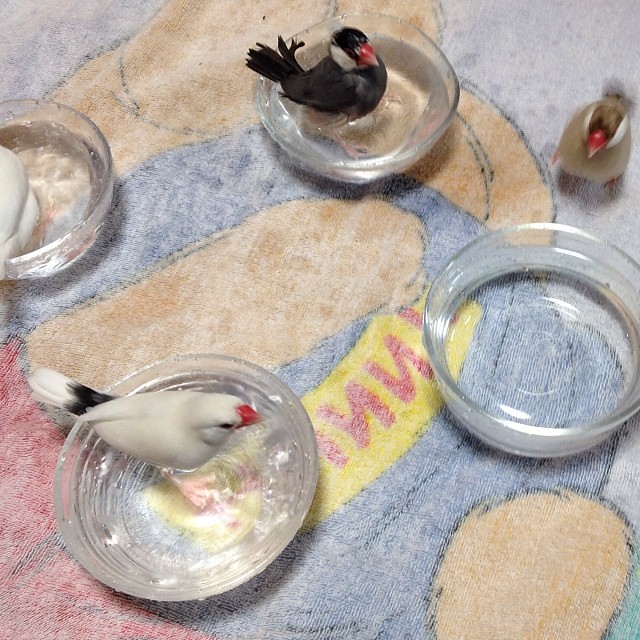This color photograph captures an overhead view of four clear bowls filled with water, arranged on a blue rug that features patterns and hints of yellow, red, and light brown. In the bottom left bowl, a striking white bird sits, its features highlighted by a red beak, black eyes, and a tail that is predominantly white with a black middle. The top right bowl holds a black bird with a reddish beak and white cheeks, contrasting its dark body. Both these birds face towards the left. There’s a third bowl at the top left corner where one can partially see a white bird, though its full form isn't visible. The fourth bowl, situated towards the center, is empty, but adjacent to it on the rug, a bird with a tan body, white neck, red beak, and tan head is seen walking towards it. The setting appears serene, with the birds gently dipping their toes into the water, creating a harmonious and tranquil scene.